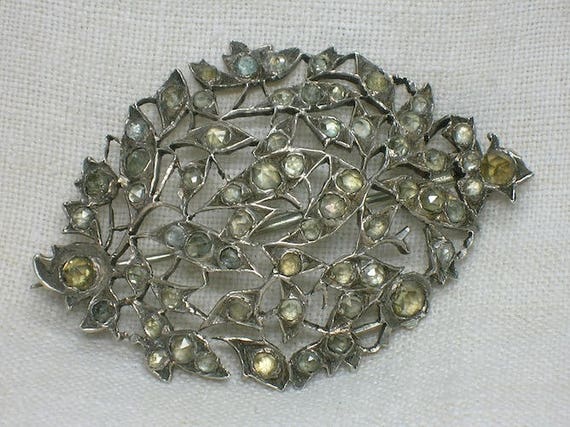This image showcases an antique-looking silver brooch or pin, intricately designed to resemble a wreath or a collection of interconnected leaves and vines, forming an oval, almost football-like shape. The brooch features decorative indentations and a variety of small, colored glass stones or rhinestones, including shades of green, brown, clear, yellow, and amber. Many of these stones are missing, adding to the brooch's aged and tarnished appearance. The brooch is quite substantial, measuring approximately four inches in width and height, and has a prominent straight pin running through it for fastening. The entire piece is captured against a light gray or blue woven fabric background, providing a contrasting backdrop that highlights the detailed craftsmanship of the brooch.